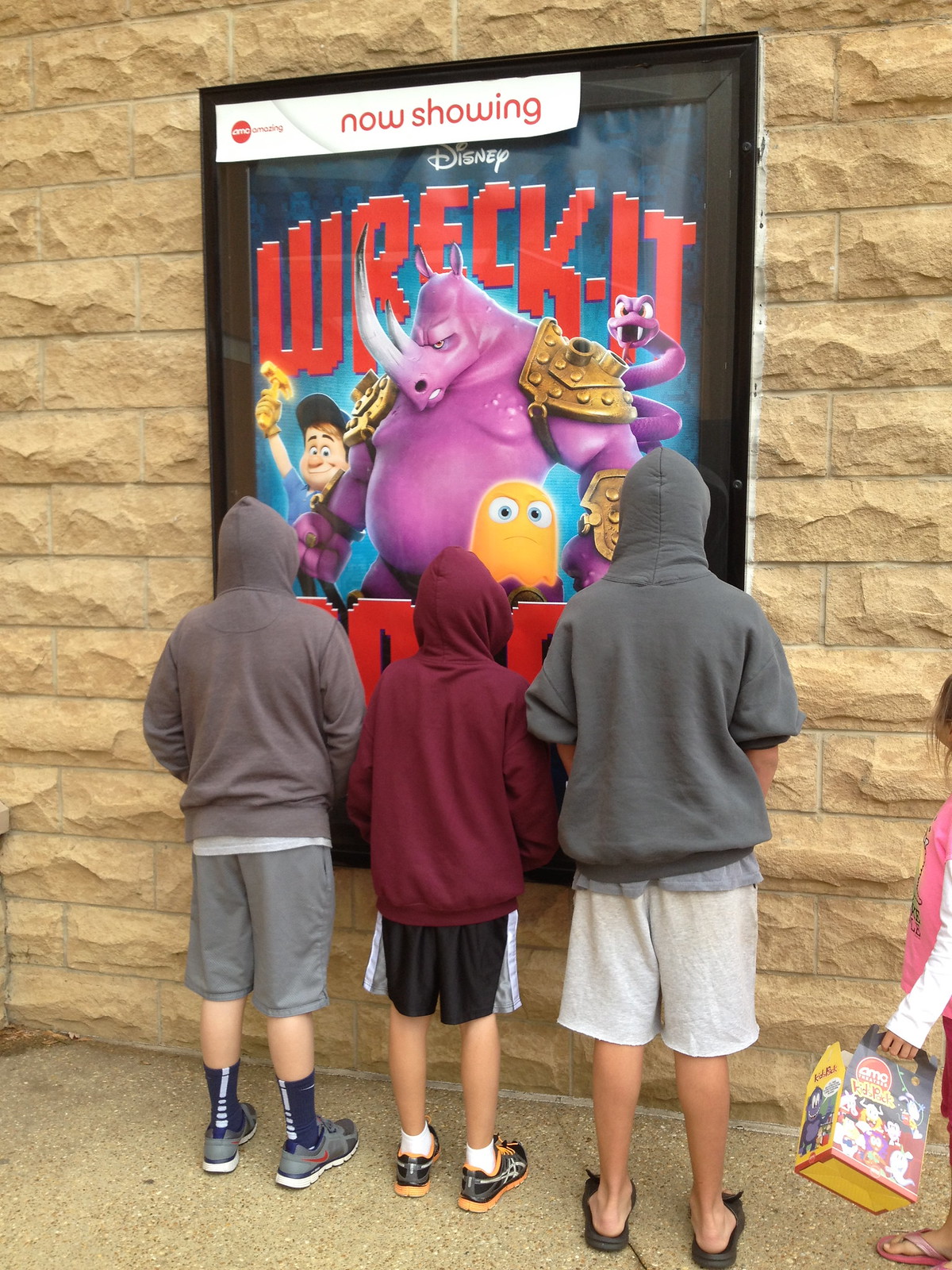In this image, three boys are standing directly in front of a large movie poster mounted on a tan-colored stone brick wall, likely the side of a building. The backdrop features a stone sidewalk, suggesting an outdoor setting, likely in the middle of the day and just outside a movie theater. The centrally positioned AMC sign is brightly colored and bears the text "AMC Amazing, Now Showing, Disney Wreck-It Ralph."

The three boys have their backs to the camera. The boy on the left wears a gray hoodie with the hood up, gray shorts, blue socks, and running shoes. The middle boy is dressed in a maroon hoodie with the hood up, black shorts with white trim, yellow ankle socks, and black shoes with white detailing. The boy on the right dons a gray hoodie with the hood up, white shorts, and open sandals without socks. 

Adjacent to them, there is a younger girl on the right side holding an AMC basket in her left hand while wearing pink slides. The movie poster itself, encased in a glass frame, features characters from "Disney Wreck-It Ralph," including a purple monster with yellow arm bands, a purple snake, a boy with a cap holding a golden hammer, and a small yellow ghost at the front. The colors present in the image range from tan, gray, dark blue, white, red, yellow, orange, pink, maroon, to purple.